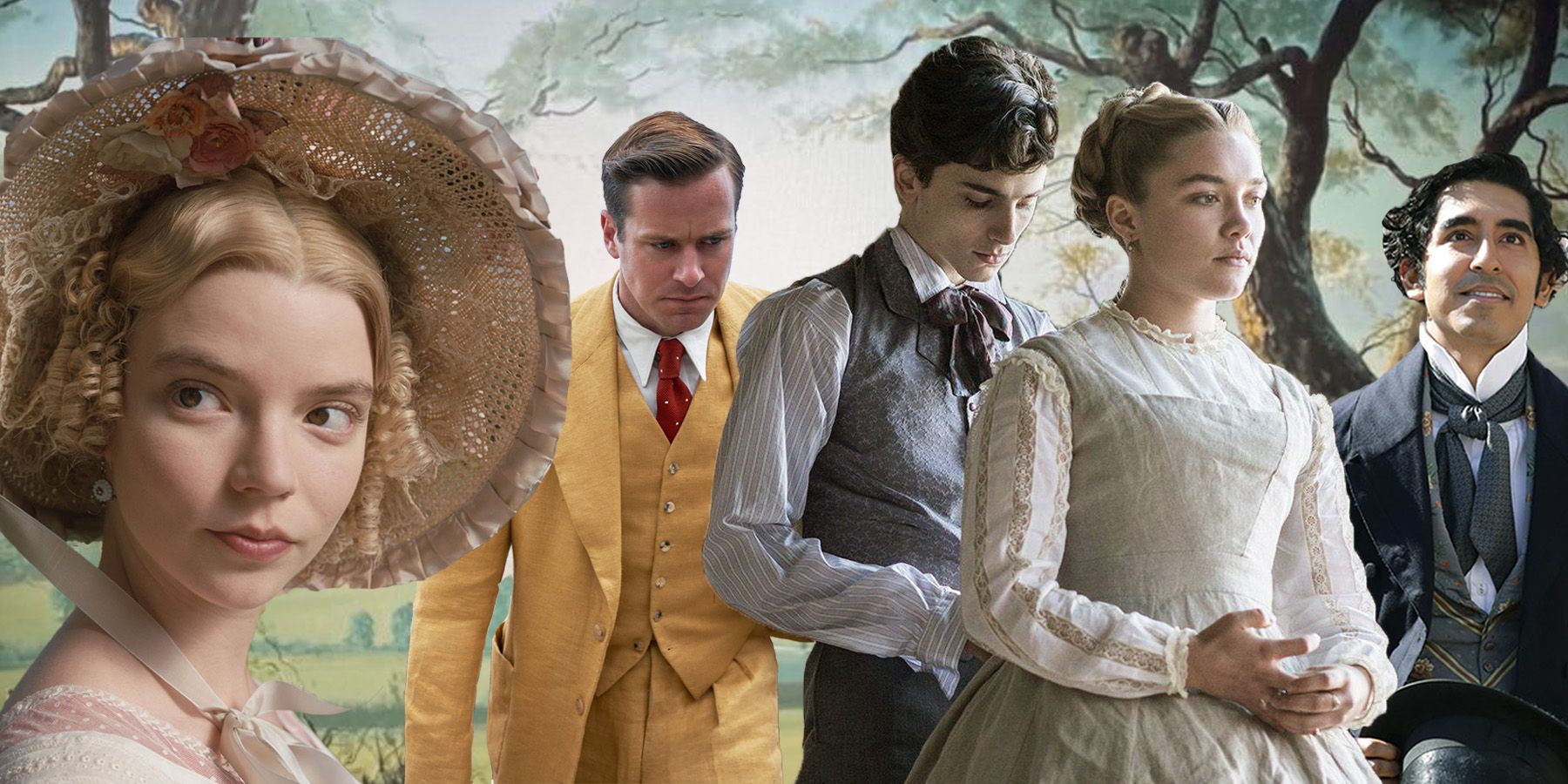This rectangular image, reminiscent of a movie cast from an 1800s period piece, features five individuals aligned horizontally. On the far left stands a woman, likely Anya Taylor-Joy, sporting short blonde hair, parted in the middle, and a wide-brimmed tan hat with bands. She wears a white lace top visible at the shoulder, red lipstick, and gazes to the left while facing the viewer. To her right is a man in his 30s, dressed in a mustard-colored suit, a white collared shirt, and a red tie. He has medium-length brown hair and his body is turned slightly to the right, with his head looking down. Next to him is a younger man with medium-length dark hair, wearing a gray vest over a white shirt, looking down as well. He stands behind a young woman in her teens or early 20s, with light-colored hair styled back, wearing a full-length white dress with gold stripes and gray detailing on the torso. She faces right with her hands together at waist level. On the far right is a man in a gray suit with a white shirt, darker vest, and a distinctive bow tie. He has medium-length black hair, curly, and holds a hat in his hand while looking upward, directly at the viewer. The background features a tree and a prairie, enhancing the historical, cinematic ambiance of the scene.